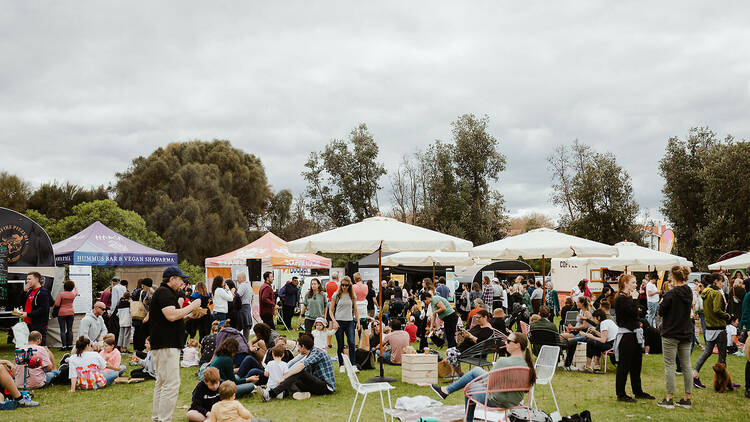This vibrant color photograph captures a large outdoor festival or concert, set in an expansive grass field bustling with hundreds of people of all ages and ethnic backgrounds. The attendees are seen either sitting on lawn chairs, standing, or walking around, creating a dynamic and lively atmosphere. In the foreground, a woman with a ponytail and shades relaxes on a pink chair near a colorful umbrella, while others nearby engage in conversation.

Scattered throughout the scene are several tents and awnings, including a blue one labeled "Hummus Bar and Vegan Shawarma," an orange and white tent, and various umbrellas providing shade. These tents and umbrellas add splashes of color against the verdant field. An ambulance and a white truck with "Budget" written on the side are visible in the background, highlighting the logistical setup of the event.

Beyond the festival area, a line of small trees with green leaves and shrubbery subtly frames the scene, beneath a thick, overcast sky, suggesting a warm but cloudy day. Despite the gray skies, the atmosphere is one of enjoyment and community bonding, as people talk and soak in the festive spirit.